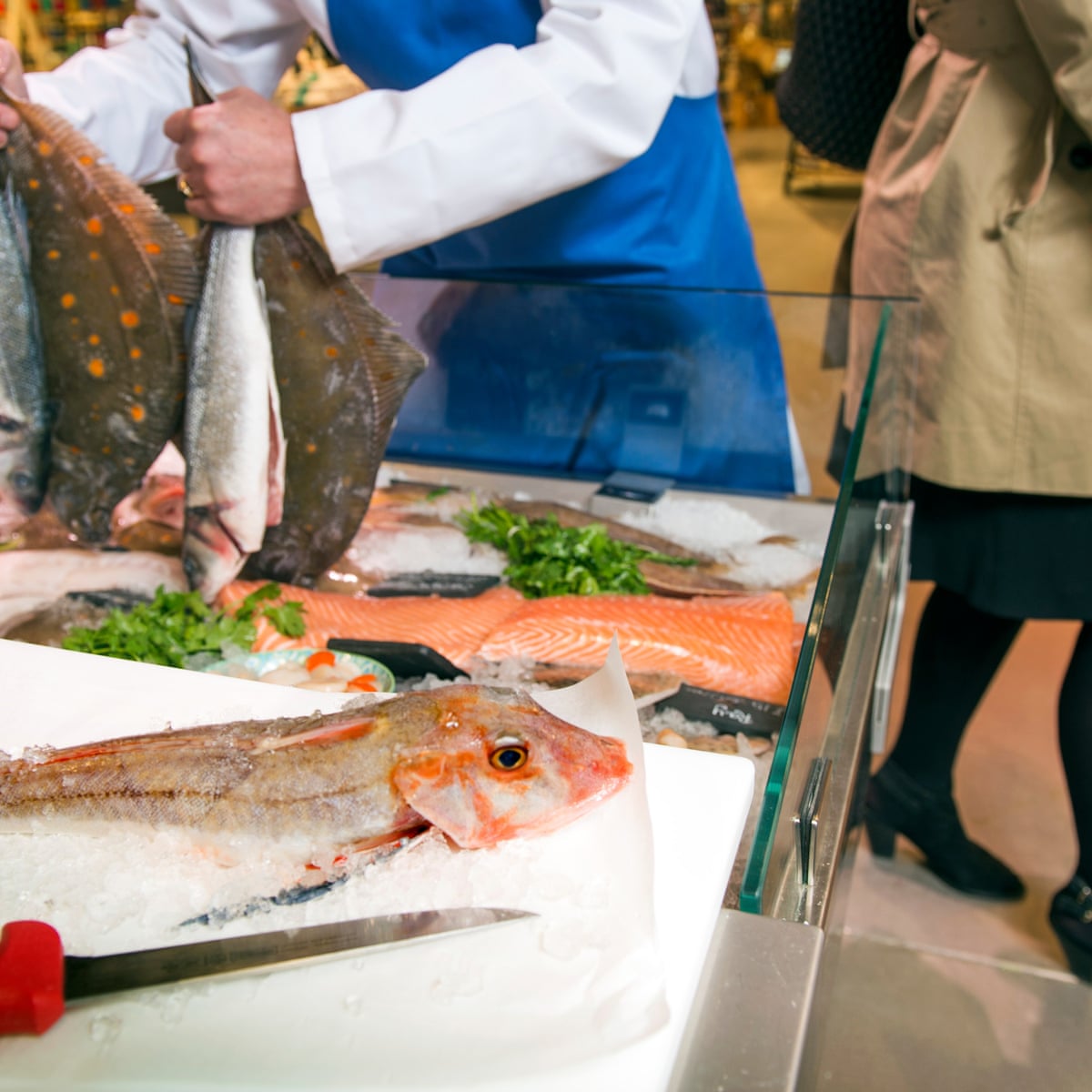The image captures a bustling fish market, likely in a grocery store or market area, where fresh fish are brought in directly from the docks. Front and center, a worker dressed in a white coat and a bright blue apron is prominently displayed. This person is holding four fish by their tails, including what appears to be two halibuts, ready to be prepared for sale. In front of him on a cutting sheet lies a freshly caught fish with ice still clinging to its skin, next to a gleaming fillet knife, ready for use. Adjacent to this untouched fish is another filleted piece, neatly presented with green vegetables. The glass display case behind them is filled with a variety of full fish and pre-prepared fillets, with a focus on salmon, indicating the freshness and variety available for customers. In the background, other market-goers can be seen walking by, adding to the lively atmosphere of the market setting.